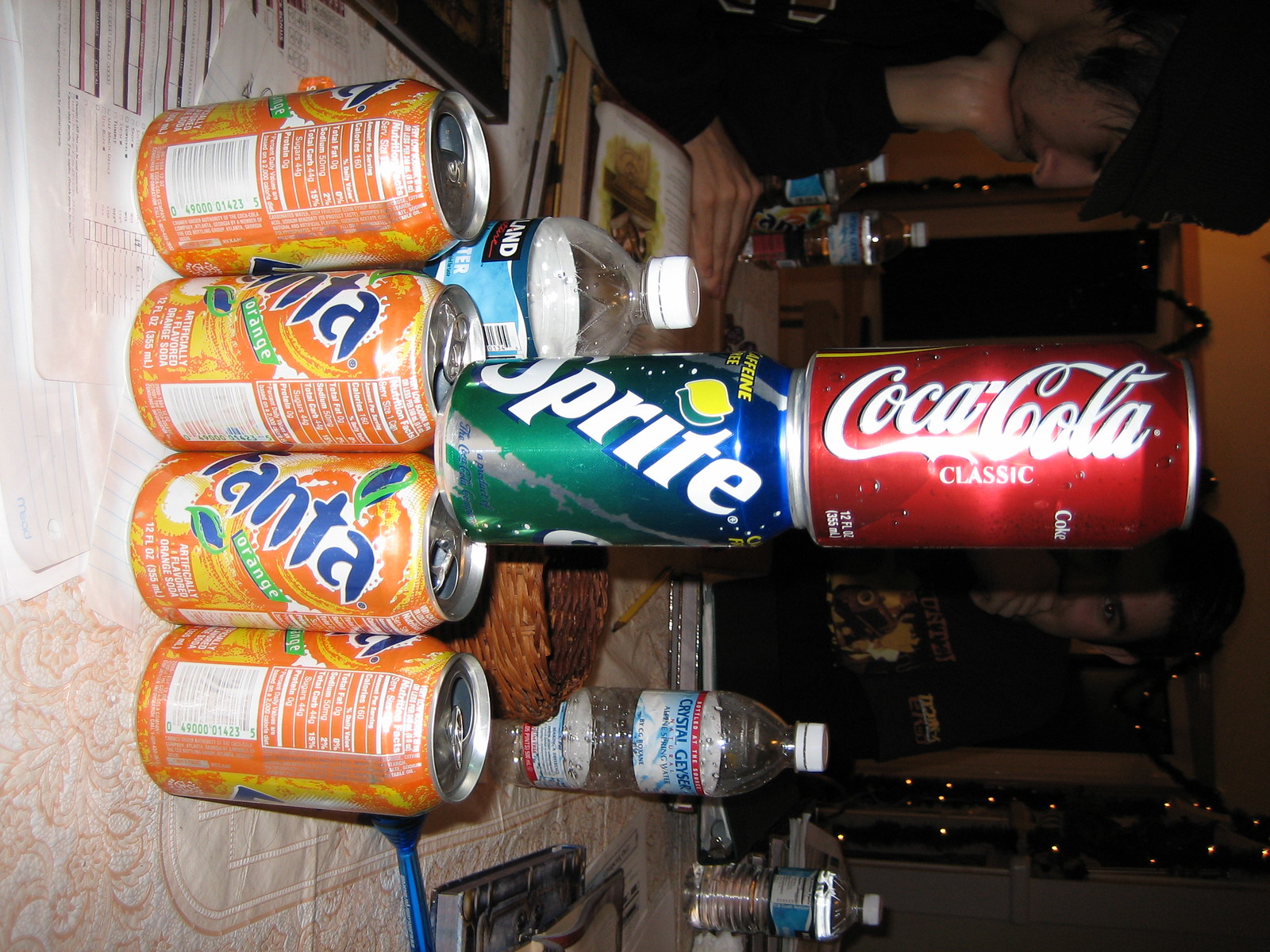A rotated, detailed photograph captures a cluttered tabletop scene featuring a meticulous arrangement of beverage cans and a surrounding mess. On the table, four Fanta cans are lined up in a row, with a Sprite can balanced on top of them, and a Coca Cola can sits atop the Sprite can, forming a tiered structure. Behind this unusual arrangement, there is a brown basket and three water bottles that resemble the texture of Crystal Geyser brand bottles. The table itself is covered with a white tablecloth and littered with numerous papers. In the background, two individuals are visible: one is absorbed in reading a book while wearing a black t-shirt and black cap, and the other is looking directly at the camera, also dressed in a black t-shirt. The scene exudes a chaotic energy, with both the table and the background filled with various items, underscoring a need for tidiness.